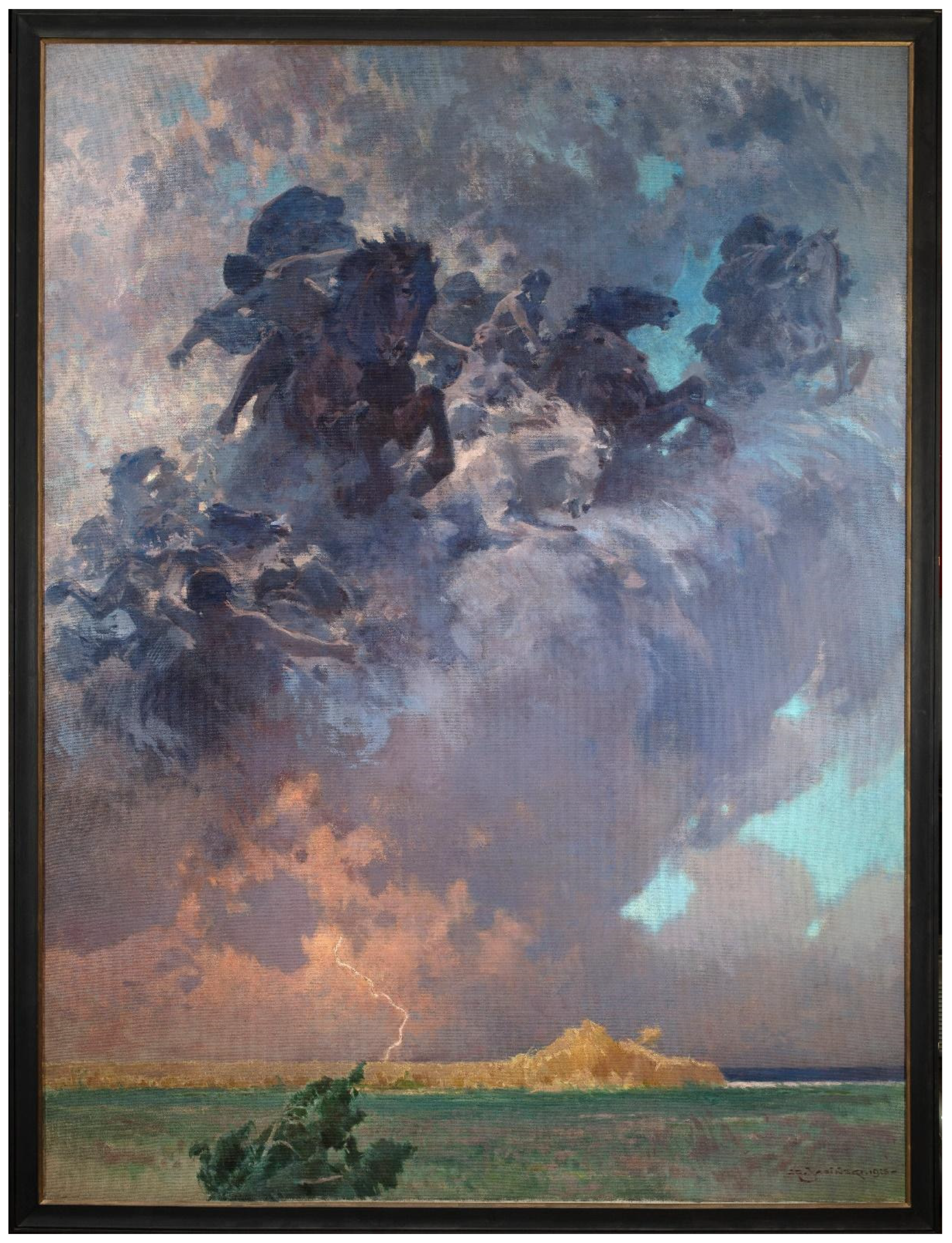This vertically rectangular painting, framed with a black border and a thin gold line, artistically depicts a dramatic sky filled with an array of clouds in shades of gray, blue, purple, and pink. The upper portion of the image is dominated by dark, purplish-gray clouds, while light blue sky peeks through in places, shifting to lighter tones at the bottom right.

In the tumultuous clouds, a series of dynamic scenes unfold. Foremost, several horses, ridden by men, appear to emerge from the clouds. The riders, depicted in darker colors, seem engaged in combat, lunging at one another, although no weapons are visible. These cloud-formed figures evoke a sense of the Four Horsemen of the Apocalypse, with the horses and riders blending seamlessly into the cloudscape, primarily in brown, white, blue, and gray hues.

At the bottom of the painting, to the left of center, a lightning bolt strikes the ground from a light gray cloud, illuminating the scene. Below this electrifying burst, the lower part of the image transitions into a landscape with a tan, rocky formation or beach area, accompanied by blue or green water suggestive of a shoreline. To the left of this, a dark-colored horse, possibly greenish, with a rider, stands in a field-like area with hints of brown and green, possibly a depiction of a battle scene's aftermath or a war-torn landscape.

Overall, the painting captures a fantastical, war-torn sky seamlessly integrated with the land below, using dramatic contrasts and fluid transitions between the elements to create a vivid, almost otherworldly scene.